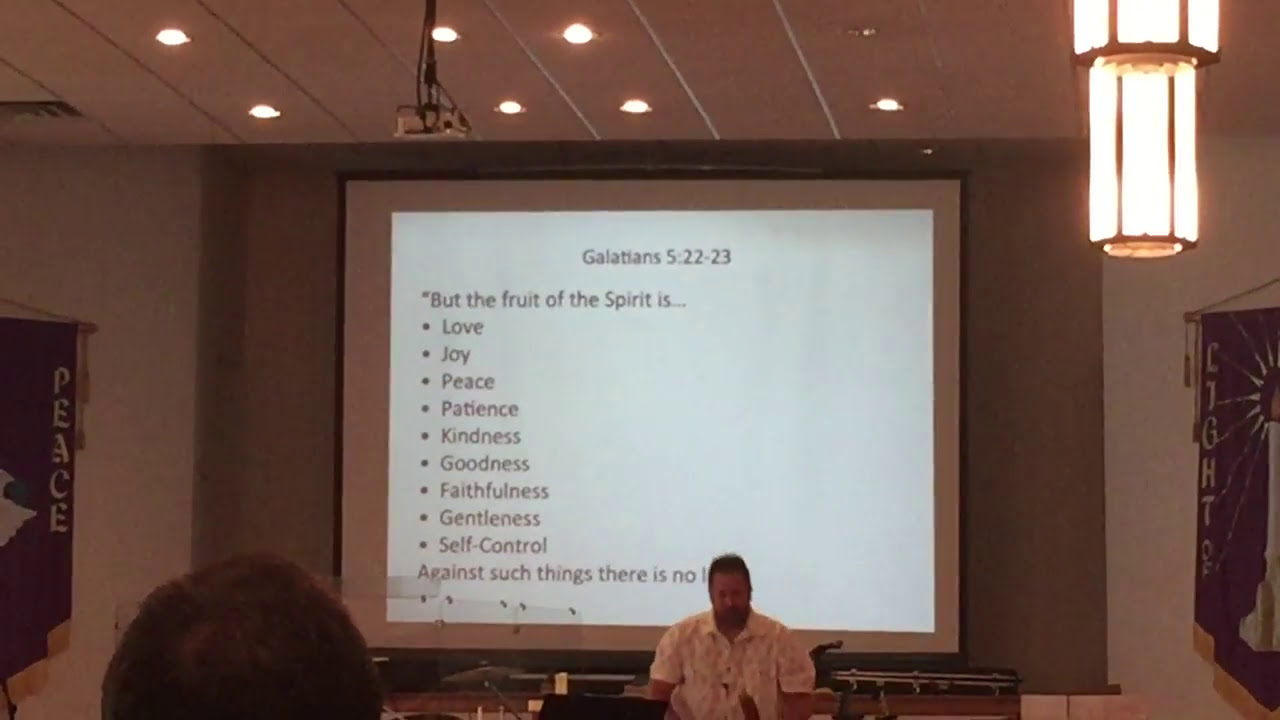This image depicts a scene inside a well-lit church or conference hall. Central to the scene is a large projection screen displaying a PowerPoint slide with the title "Galatians 5:22-23," which is a biblical verse about the Fruit of the Spirit. The slide lists virtues such as love, joy, peace, patience, kindness, goodness, faithfulness, gentleness, and self-control. The last phrase on the slide begins with "against such things there is no," but the final word is obscured by a man standing in front of the screen. This man appears to be addressing an audience, wearing a short-sleeved, collared white shirt, and has dark hair. He might be Caucasian, suggested by his light skin tone. Only one member of the audience is partly visible – a person with dark brown hair seen from behind. The room features recessed ceiling lights and a visible chandelier in the top right corner. Both the left and right sides of the wall have purple banners, reading "Peace" and "Light" respectively. The screen occupies most of the middle portion of the image and is set against a beige wall.